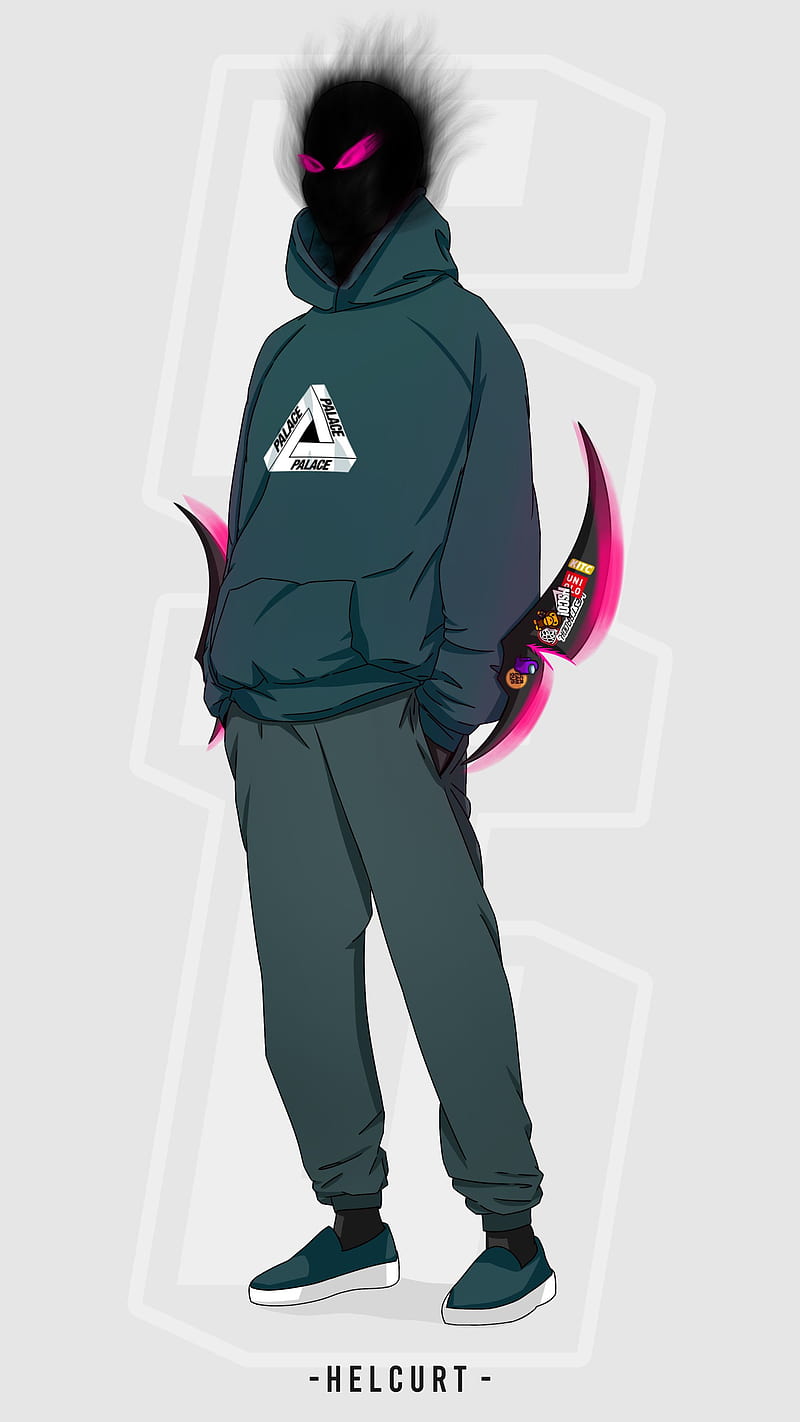This is a detailed digital artwork of a video game character named Helcurt, presented in an anime-inspired style. The character is depicted in a green hoodie featuring a distinctive triangle design with the word "palace" on each side, paired with slightly lighter green sweatpants. His footwear consists of green slip-on sneakers similar to boat shoes with white soles, complemented by black socks. Helcurt’s head is an eerie, featureless black void emanating wispy, smoky tendrils, highlighted by vivid violet eyes, giving him a sinister, demonic appearance. His arms rest casually in his pants pockets, but dual-headed blades, resembling axes or scythes with violet edges, extend from his forearms, indicating a blend of casualness with underlying menace. The name "Helcurt" is prominently displayed at the bottom of the image.